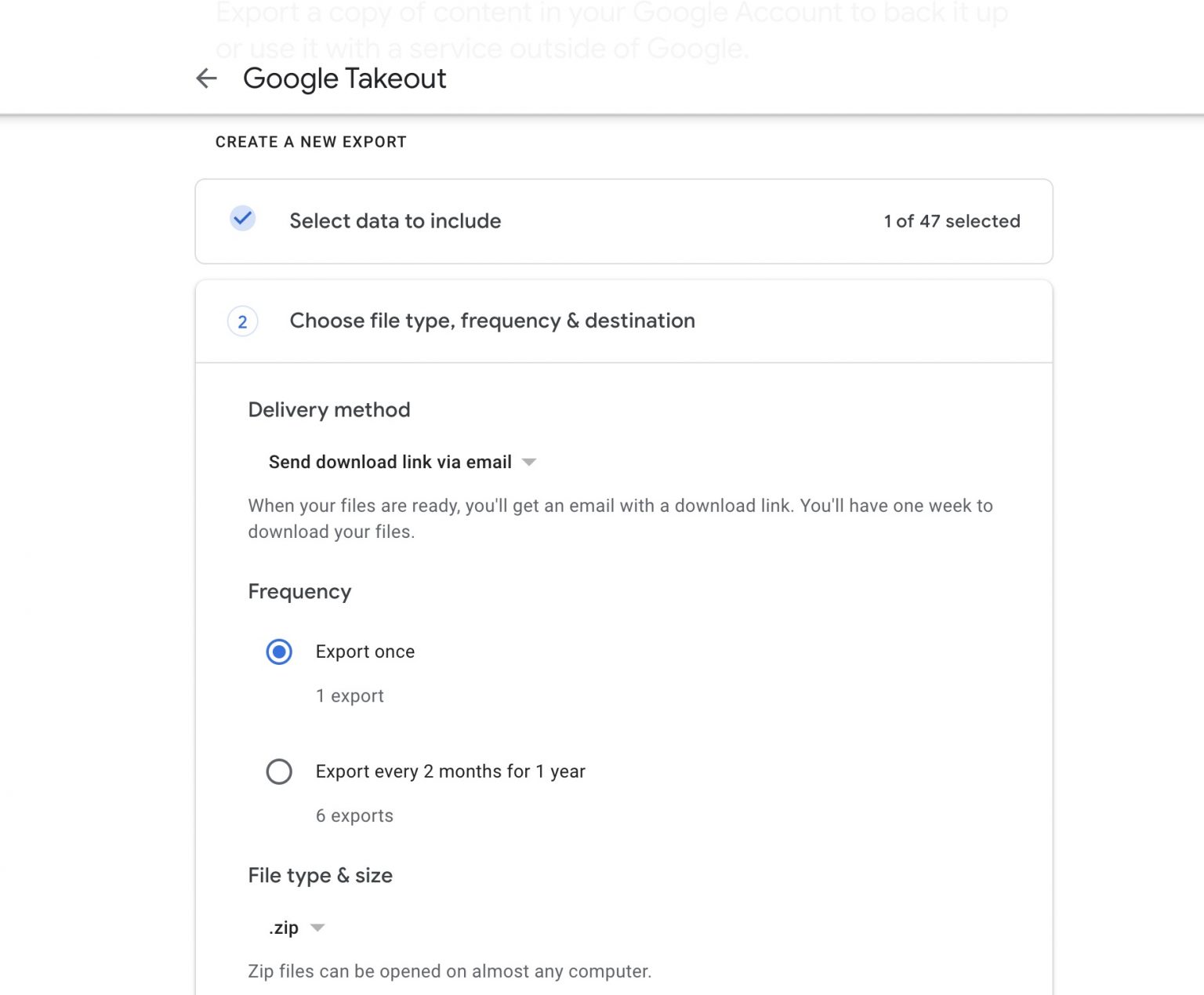In this image set against a white background, the upper-left corner features the "Google Takeout" logo with an arrow pointing left. Below a thin gray line reads "Create a new export." Beneath this, there is a box with a small blue circle and blue checkmark labeled "Select data to include," and to the right, it shows "1 of 47 selected."

The next box below provides options to "Choose file type, frequency, and destination." The delivery method is "Send download link via email." The instruction reads, "When your files are ready, you'll get an email with a download link. You'll have one week to download your files."

Highlighted in bold black text is "Frequency." The option "Export once" is circled with a blue dot, indicating it is selected. Below it, the option "Export every two months for one year (six exports)" is listed.

In another section, also highlighted in bold text, is "File type and size." Below this header, a dropdown arrow next to "zip" indicates a selectable file type.